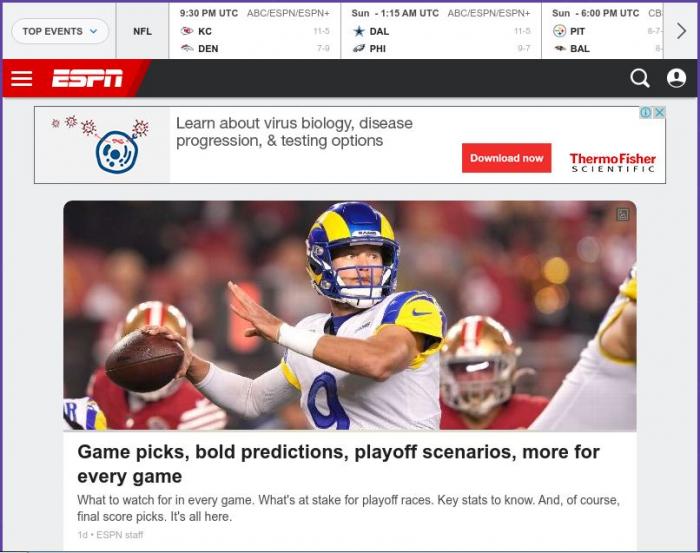**Detailed Caption:**

This is a detailed screenshot of the ESPN website, a major sports broadcaster in the United States, focusing on American football. At the top of the page, a ticker displays various sports scores and updates, commencing with the label "Top Events" accompanied by a dropdown menu. Adjacent to it, "NFL" signifies coverage of the National Football League. The ticker lists upcoming fixtures in UTC format, including a game at 9:30 PM UTC between Kansas City Chiefs (KC) and Denver Broncos (DEN), followed by another matchup on Sunday at 1:15 AM UTC between the Dallas Cowboys (DAL) and a team represented as FI, speculated to be the Philadelphia Eagles. Additionally, it lists a game on Sunday at 6:00 PM UTC featuring Pittsburgh Steelers (PITT) and Baltimore Ravens (BAL).

Beneath the ticker, a red bar prominently features the stylized ESPN logo, with all letters aligned to equivalent height. Below this, a narrower black bar holds a search icon and a user login icon. An advertisement banner from Thermo Fisher Scientific follows, promoting educational resources on viruses, biology, disease progression, and testing options, with a downloadable option.

The central content is a news story headlined "Game Picks, Bowl Predictions, Playoff Scenarios, More for Every Game." Accompanying the headline is an image of an American football player wearing a blue and yellow striped helmet and a white jersey with blue and yellow accents on the shoulders, bearing the number nine. He is seen carrying a football, with background players adorned in red uniforms and gold helmets marked with red and white stripes. The article delves into what to watch for in each game, playoff implications, key statistics, and final score predictions.